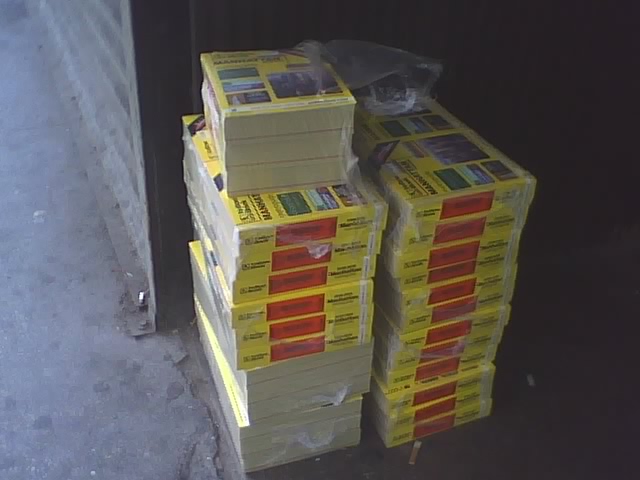The image features four neatly arranged stacks of thick phone books, each carefully wrapped in clear cellophane, indicating they are new and awaiting distribution. The stacks are positioned diagonally, with one stack in front of the camera and another directly behind it, forming two rows of two stacks each. The prominent yellow spines, with conspicuous red blocks in the center showcasing black text, highlight the branding and possibly advertising material. The visible covers are adorned with promotional images likely indicative of the city they serve, although the text is too small to decipher the specific location. Each phone book is about two inches thick. The stacks on the right side of the image contain phone books uniformly aligned, with the yellow and red spines consistent throughout. The ground below is a dull concrete gray, and a small portion of the wall on the left is visible, displaying a similar grayish tone, while the right side recedes into darkness. Notably, there is a cigarette butt discarded in front of the stacks on the right, adding a touch of everyday realism to the scene.